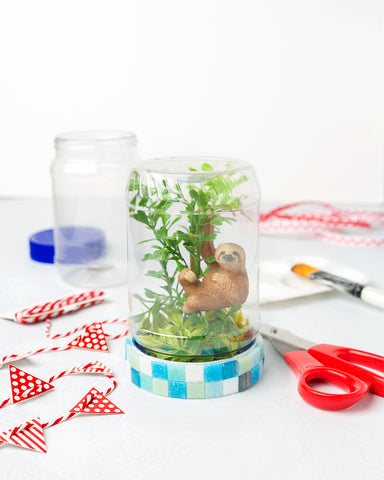On a white tabletop with a white background, the image showcases a diverse array of craft supplies arranged meticulously. The central focus is an upside-down jar with a blue, green, and white mosaic base, detailed with intricate small tiles. Inside the jar sits a charming plastic sloth clinging to a miniature branch surrounded by fake green foliage, evoking a playful scene of nature. Red-handled scissors are neatly placed inside the jar, adding to the artistic setup.

In the background, an upright jar with its blue lid removed is partially visible. To its right, a paint palette is accompanied by a white paintbrush with a silver ferrule and yellow bristles. Enhancing the lively crafting environment, a vibrant banner of red triangles is threaded with a red and white candy-cane-striped string, with alternating patterns of polka dots and stripes. Additional red and white twine can be seen winding through the scene, emphasizing the festive and meticulous crafting session that the image captures.